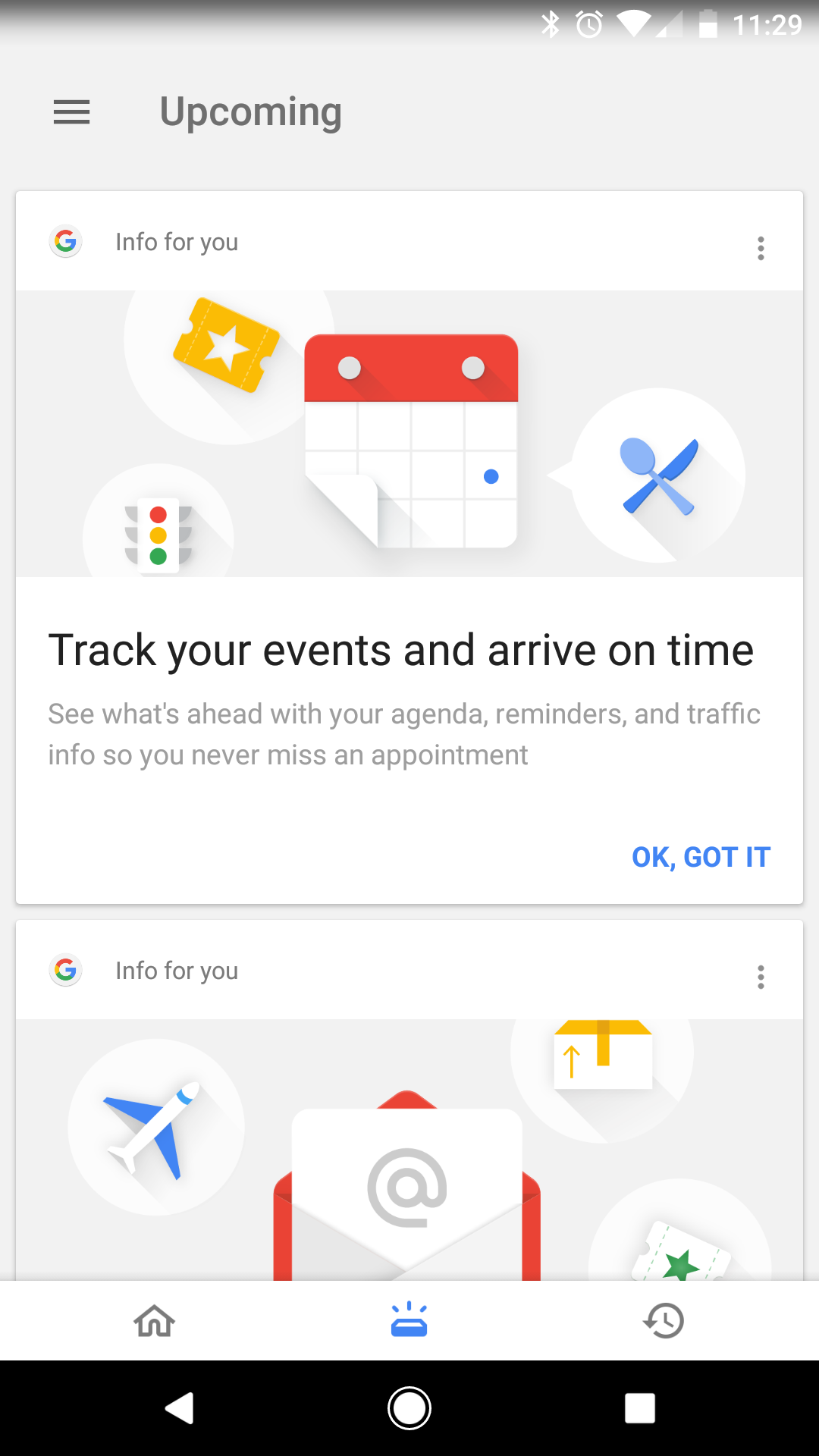In this screenshot of an Android mobile device, we observe various status icons located in the top-right corner. These icons display the Bluetooth connection status, an active alarm, Wi-Fi signal strength, cellular network signal strength, battery level, and the current time, which is 11:29. Below these icons, there is a prominent search field labeled "Info for You." Further down the screen, informational text highlights the device's capabilities, such as tracking events, sending reminders, and providing traffic information to ensure timely arrivals for appointments. The user is prompted with the message "Okay, got it." At the bottom of the screen, the standard Android navigation buttons are visible, including options to go back, return to the home screen, and view recent applications.